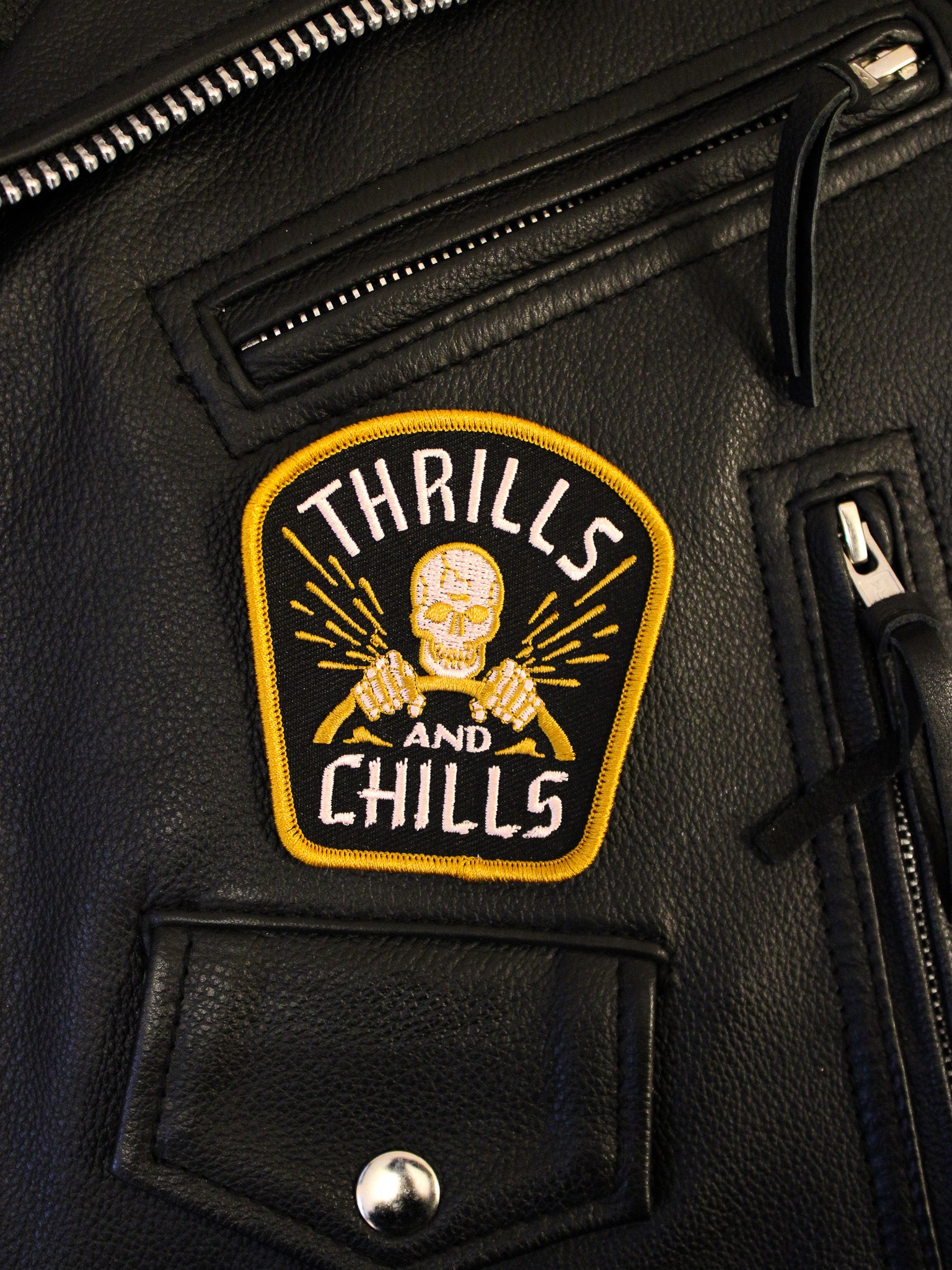This close-up photograph showcases a section of a black leather motorcycle jacket adorned with various intricate details. Central to the image is a patch sewn onto the leather, shaped with a flat bottom and a curved top edge, outlined in gold thread. The patch features a black background with the word "THRILLS" embroidered in white capital letters at the top. Below this is a detailed illustration of a skeleton, its skull and bony hands emphasized with white and gold stitching. The skeleton grasps a steering wheel, with yellow streaks emanating from both sides. The words "AND CHILLS" appear in white below the skeleton. Directly underneath the patch, there's a leather pocket secured by a silver button, with a vertical zipper to its right. Additionally, another zipper runs horizontally above the patch on the right, and the upper left corner of the image reveals the teeth of yet another zipper. The meticulous craftsmanship and the assorted zippers contribute to the jacket's rugged aesthetic, making it a striking piece.